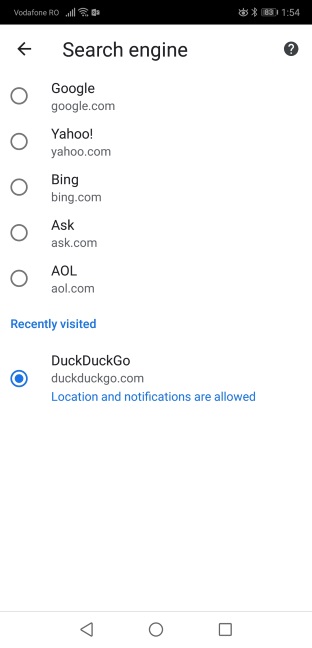A screenshot of a phone is displayed on a website. The phone shows the time as 1:54, with the battery critically low at 3%. The carrier name "Vera Verda" appears in the upper left-hand corner next to other status icons. At the top of the screen, there are large, bold letters that say "Search Engine". An arrow pointing left is positioned below, alongside a circular icon with a question mark on the right.

The main section of the screen lists various search engine websites next to hollow circles. The websites listed are:
1. Google (google.com)
2. Yahoo (yahoo.com)
3. Bing (bing.com)
4. Ask (ask.com)
5. AOL (aol.com)

Below this, in blue text, it shows "Recently Visited" with the website DuckDuckGo (duckduckgo.com). Next to DuckDuckGo, the circle is filled in blue, indicating it is selected.

Towards the bottom of the screen, phrases in blue state that "Location and notifications are allowed." The rest of the screen is filled with white space down to the phone's standard navigation icons at the bottom.